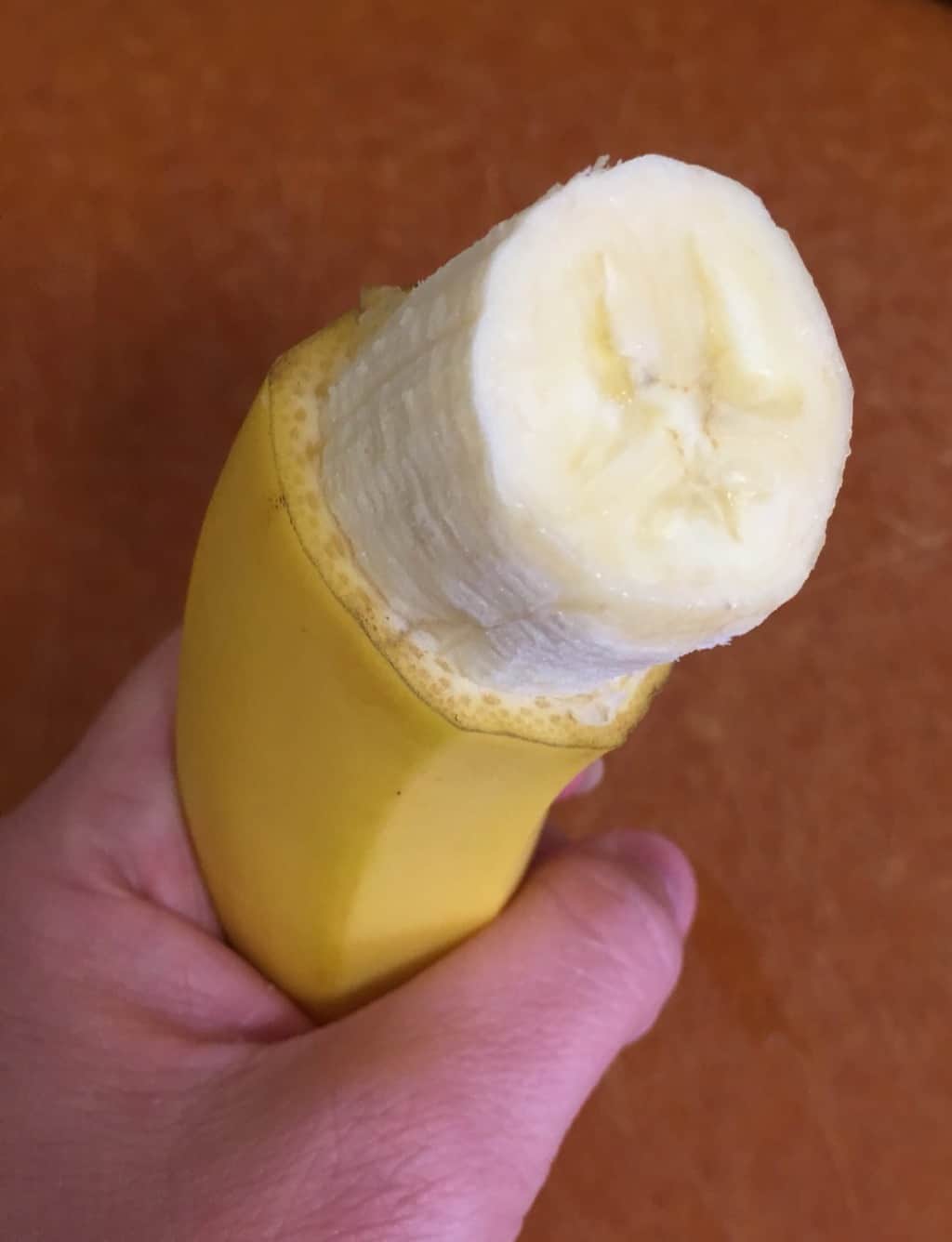A close-up photograph captures a person's left hand, with a visible beige thumb and thumbnail, holding a partially peeled banana in a manner resembling an ice cream cone. The banana, prominently centered, bends towards the upper right corner. Its light yellow flesh, which appears either bitten or sliced off, contrasts against the remaining skin still attached at the bottom. The peel is perfectly edged off, showcasing a bit of the porous texture. The background is a solid brown with a hint of white, possibly indicating a wall, floor, or countertop, forming a monotone backdrop that accentuates the dramatic presentation of the banana.